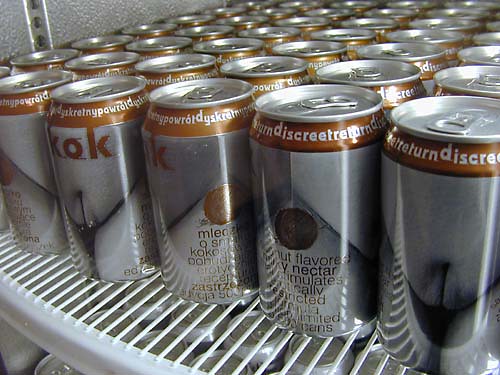The image depicts the inside of a refrigerator, featuring a white metal rack with several rows of neatly lined silver cans. The rack has thin white beams stretching across it, and the shelf is visible in the bottom left corner. Each can showcases a distinct design, including a bronze or copper-colored trim around the top, and white text that appears to read "discrete." The cans feature a black half-circle at the bottom and illustrations that seem to portray the groin area of an overweight person, emphasizing the belly button. The cans are designed with a combination of silver, black, and white hues, and the tops of the cans, equipped with pull tabs, are also silver. There are at least six rows of cans visible, extending further back into the cooler. Through the grates of the shelf, the tops of the cans can be clearly seen, highlighting their uniform alignment.